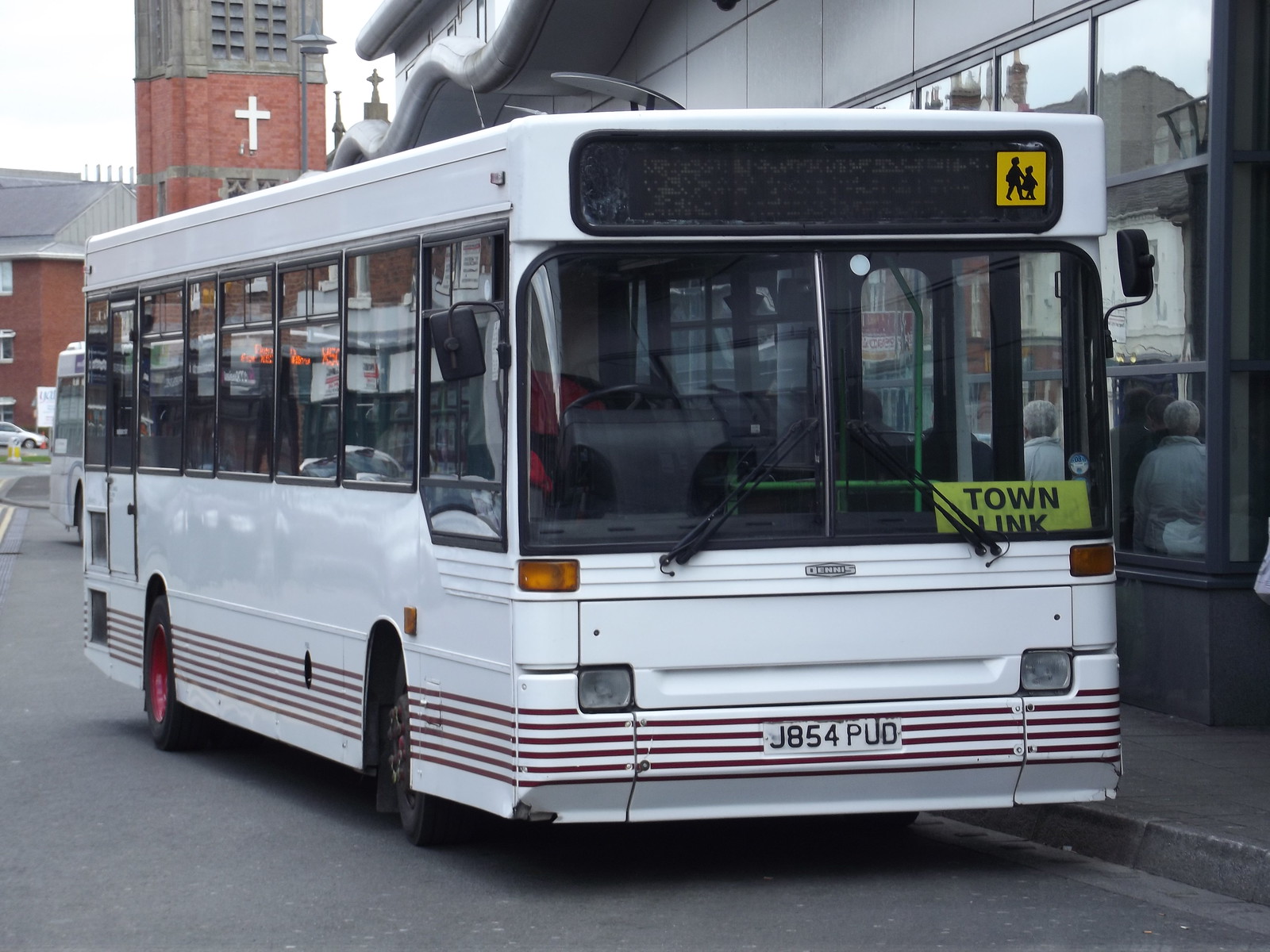The photograph features an older white transit bus, parked on the side of a gray or blacktop road, likely next to a bus depot characterized by a dark gray building with long, front-facing windows and a corrugated metal roof. The bus is viewed slightly from an angle, with the front facing the camera. The bus has a large windshield at the front, extending upwards, with windows running along its entire side. In the lower right corner of the windshield, there's a yellow sign with black print that reads "Town Link." Above the windshield is an empty digital sign for destination display. The license plate, J854 PUD, is visible on the lower grille of the bus.

In the background, behind the bus, stands a large old church made of reddish-brown bricks. This church features a prominent steeple with a white cross and large front tower. Reflections in the bus windows and those of nearby buildings include people standing. The image contains a mix of colors including white, yellow, black, gray, reddish-brown, silver, and orange. The setting is an outdoor, daytime scene in a likely urban environment, possibly a European city.